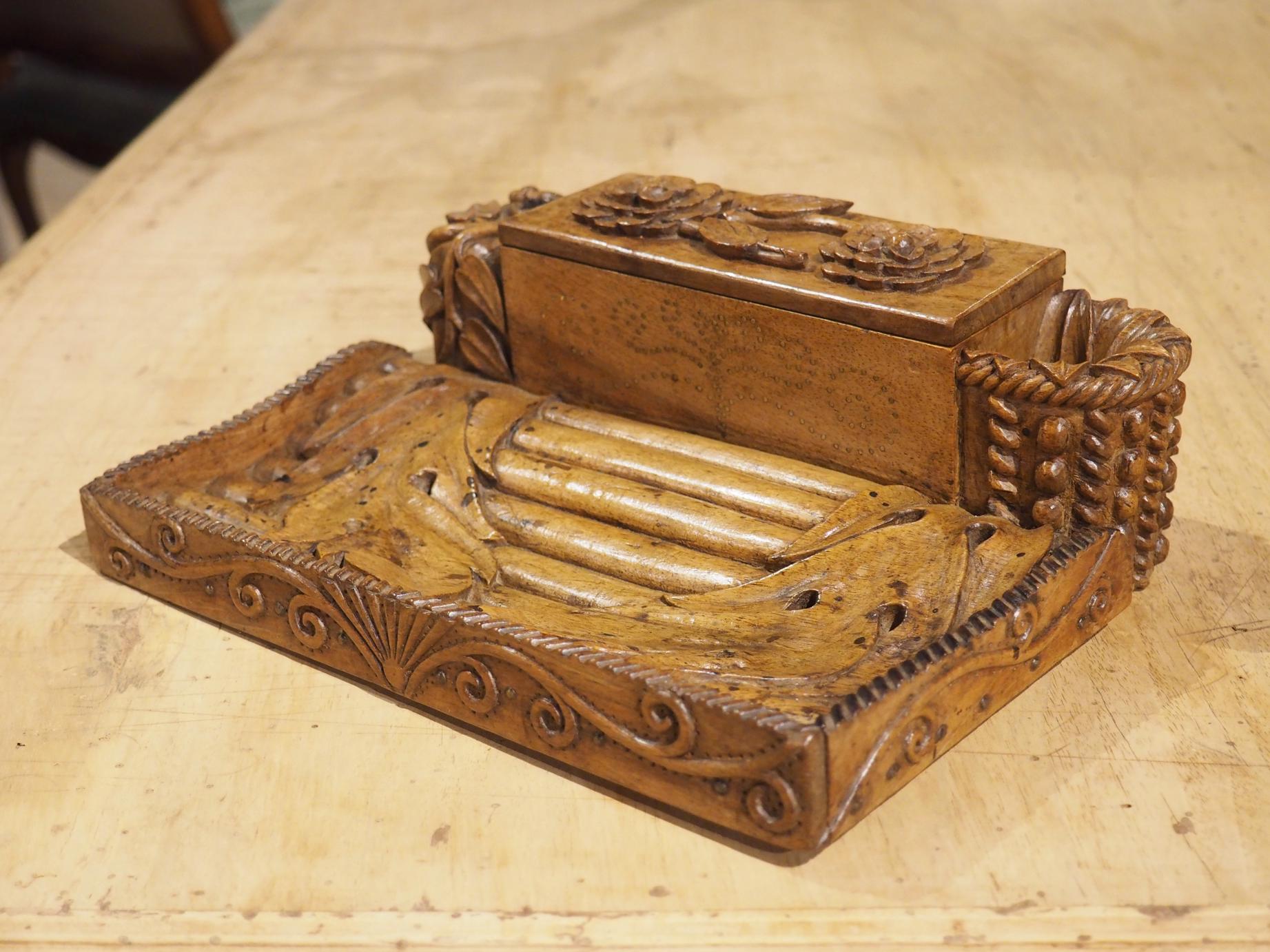The photograph showcases a beautifully ornate, vintage wooden box set against a light wood table that fills the background. The box, crafted from light, blondish wood, is meticulously carved with intricate designs. The lid of the box features carved leaves and flowers, possibly reminiscent of Pennsylvania Dutch or early American style motifs. On the front, a rectangular compartment displays elaborate carvings, including swirling curlicues and relief patterns. On the right side, a semicircular compartment with rope-like detail and rosettes complements the main box. Below, a tray-like base is adorned with a sawtooth rim and designs resembling rolled pieces of wood or cigars, bordered by swirly lines. The large flat object, potentially a lid or separate section, adds to the antique charm with its carved tobacco-like leaves, making the overall piece appear to be a unique combination of a storage and decorative wooden item.